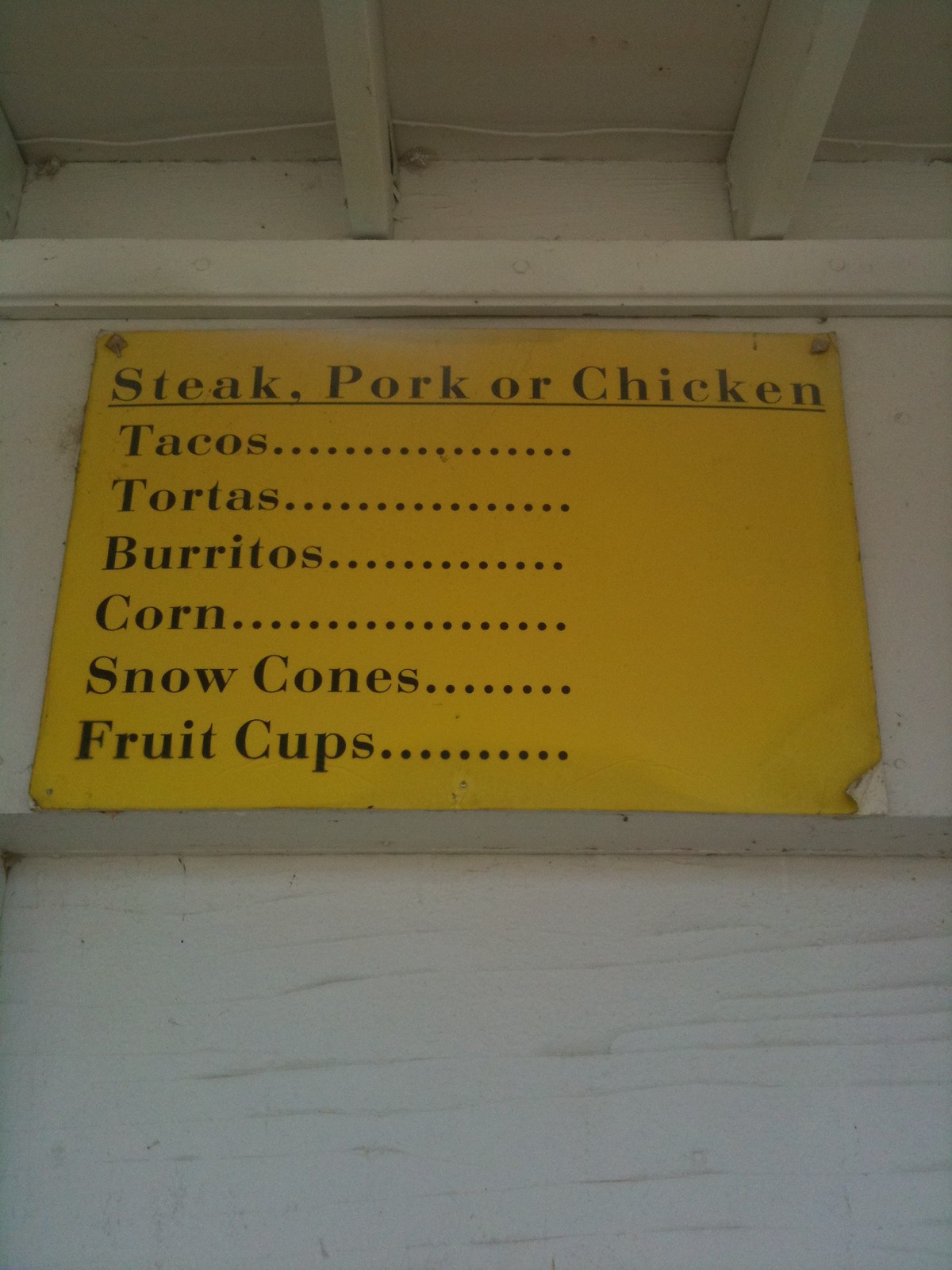The image depicts an interior wall and ceiling section. The wall has a gradient of tan shades, with a lighter tan near the top transitioning into a darker tan towards the bottom. The wall features wooden elements, adding a rustic touch to the scene. Near the ceiling, there are light gray horizontal bars, and below these, there is a lighter gray wooden beam. Underneath this beam, a darker gray section is visible, continuing the color theme.

Affixed to the wall is an orange sign that appears to be slightly worn, particularly torn at the lower right-hand corner. The sign lists various food items in black text: "Steak, Pork, or Chicken" is written at the top, underlined by a black line. Following this are the words "Tacos...", "Tortillas...", "Burritos...", "Corn...", "Snow Cones...", and "Fruit Cups...", each followed by several dots. Below the sign, the wall transitions into a slightly darker gray shade with some lighter gray lines interspersed within it, adding to the textured look of the wall.